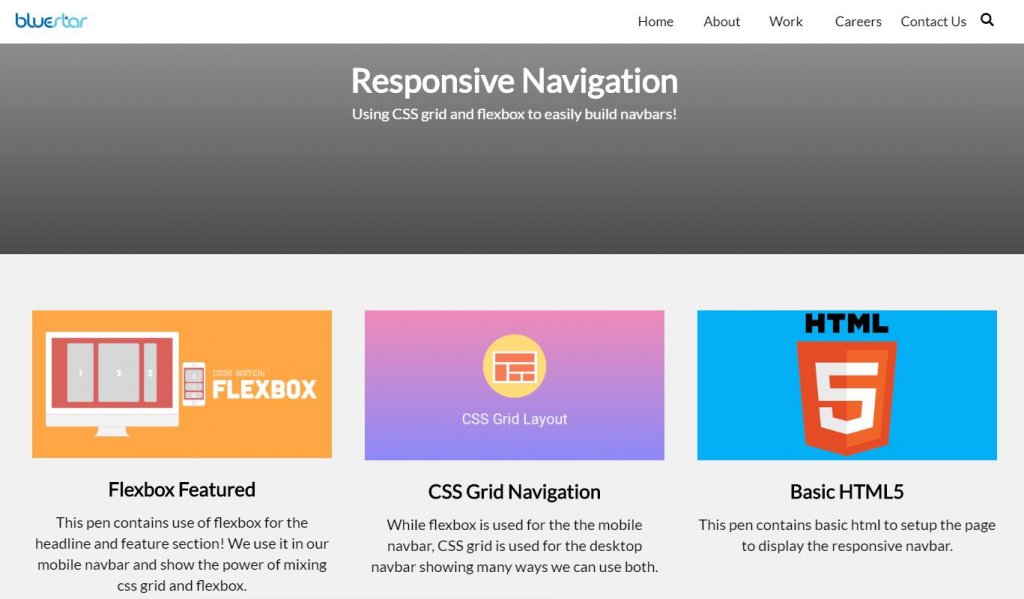A detailed and clean caption for the given image could be:

"The image displays a section of the Blue Star website. Prominently featured in the top left-hand corner is the Blue Star logo. On the top right corner of the webpage, there are five distinct menu options labeled Home, About, Work, Careers, and Contact Us, accompanied by a magnifying glass icon for search functionality. Below the navigation bar, a large gray box occupies about one-third of the screen's height, with white text centrally aligned within it. The main header within this box reads 'Responsive Navigation,' and underneath it, a subheader states, 'Using CSS Grid and Flexbox to Easily Build Nav Bars.' 

Beneath this introductory section, three smaller images are displayed. The first image depicts a computer screen and tower next to an orange box labeled 'Flexbox Feature.' The accompanying text explains that this feature demonstrates the use of Flexbox for the headline and features section, as well as for the mobile navigation bar, highlighting the combination of CSS Grid and Flexbox.

The second image showcases a purple box labeled 'CSS Grid Layout.' The text here notes that while Flexbox is employed for the mobile navigation bar, CSS Grid is utilized for the desktop navigation bar, illustrating multiple methods of integrating these technologies.

The final image is an HTML5 icon labeled 'Basic HTML5.' The description clarifies that this section contains basic HTML setup necessary to display the responsive navigation bar."